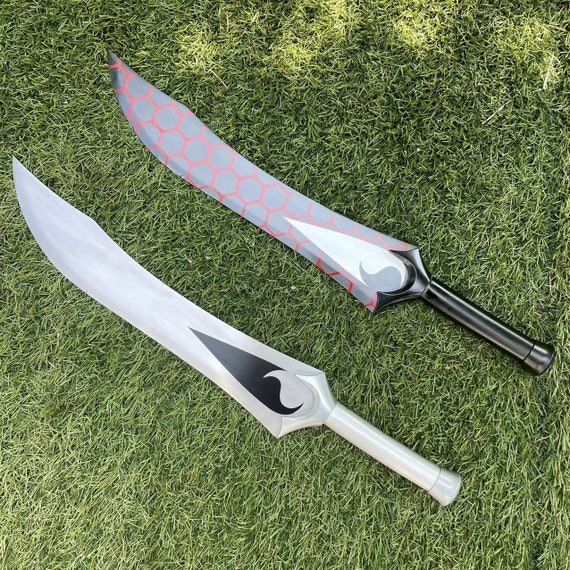The image depicts two broad, curved fantasy swords resting on a neatly trimmed or possibly synthetic green lawn. The bottom sword features a predominantly silver blade with a distinctive black triangular mark at its base, shaped like a smaller blade, and is equipped with a reflective, white handle. The upper sword possesses a black handle and a primarily black blade enhanced by a striking red hexagonal pattern that accentuates its length, reminiscent of beehive structures. Both swords give off an exotic, almost scimitar-like vibe, though they appear to be decorative models, likely from a cosplay event or fantasy collection, rather than functional weapons, and notably lack guards.